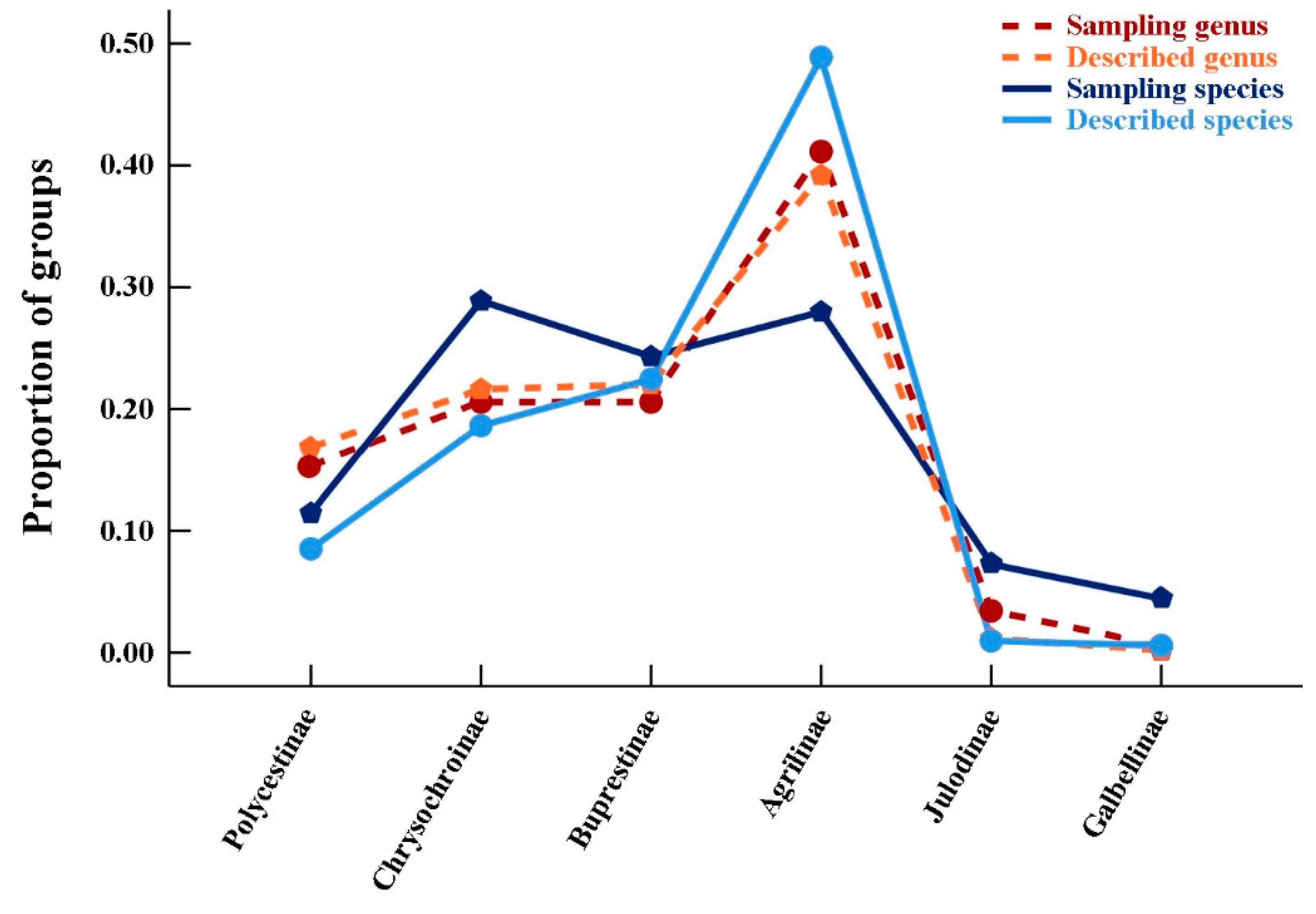The image is a detailed screenshot of a line chart displayed on a white background. The chart has a vertical y-axis labeled "Proportion of Groups," incrementing in decimal places from 0.00 to 0.50, and a horizontal x-axis labeled with the names of different groups: Polycystinae, Chrysochronae, Buprestinae, Agrylinae, Judinae, and Gabylinae. 

The chart contains four distinct lines, each represented in different colors and styles to indicate different data types, as specified in the legend located at the top right of the chart. A red dotted line represents the sampling genus, an orange dotted line represents the described genus, a solid dark blue line represents the sampling species, and a solid light blue line represents the described species. 

The data trends show varying proportions across different groups. Notably, the Agrylinae group exhibits the highest spike in proportions, nearly reaching the 0.50 mark for multiple lines. In stark contrast, the Judinae and Gabylinae groups have the lowest proportions, approaching almost zero. This chart appears to be part of a research paper or scientific article, meticulously illustrating the distribution and comparison of sampling and described genera and species across several taxonomic groups.